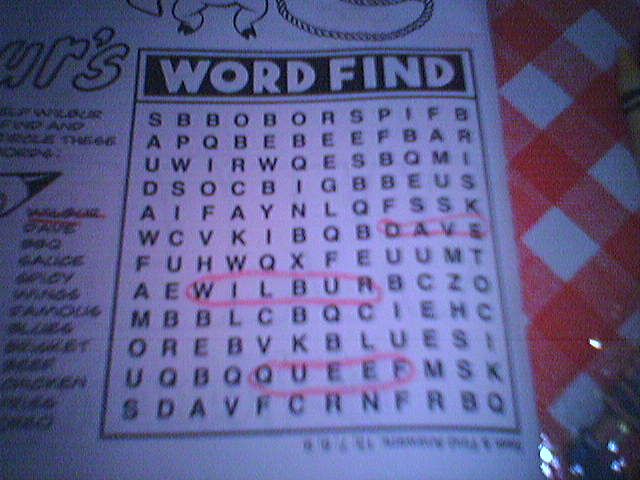The image is a photograph of a white booklet page, likely from a family restaurant's activity book for children. It was taken in a dimly lit environment, which casts a shadow over the page, giving it a dark appearance. Central to the image is a word finder puzzle, featuring an array of letters in a square grid, with several words circled in red crayon. The circled words include "Dave," "Wilbur," and "Queef." Additionally, there are other words within the puzzle like "BBQ sauce," "spicy," "wings," "famous," and "chicken," though the clarity declines towards the bottom left of the image. Above the puzzle, partially cropped out, are the hooves of what appears to be a pig, and a circular lasso rope. The booklet is placed on a table adorned with a red and white checkered tablecloth, and a partially visible yellow crayon appears at the top right. This setting, with the red crayon circles and the casual ambiance, suggests a playful, family-friendly environment.